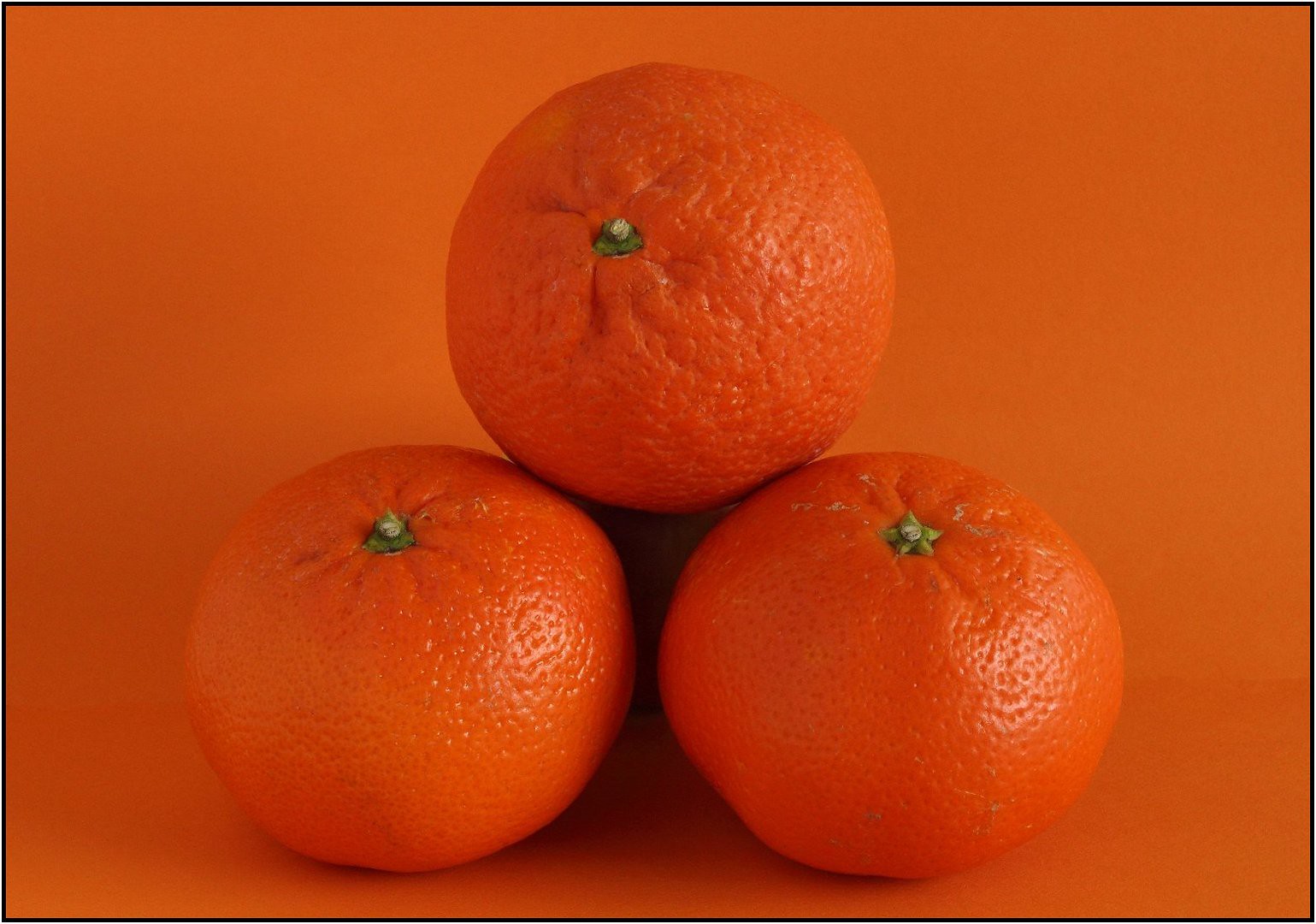This image features three medium-sized oranges arranged in a pyramidal or triangular formation, with two oranges at the bottom and one positioned on top. The oranges are a deep, vivid orange color that contrasts subtly against an entirely orange background. Their surfaces exhibit small indents and a slightly wrinkly texture, with white highlights reflecting off their shiny skins, suggesting a light source from the right side. Each orange has a tiny, greenish-beige stem at its top, resembling a star, adding a distinctive detail. Dark shadows beneath the stacked oranges accentuate their three-dimensionality, further highlighted by the mostly orange, monochromatic setting that gives the oranges a blending yet distinctly vibrant appearance.